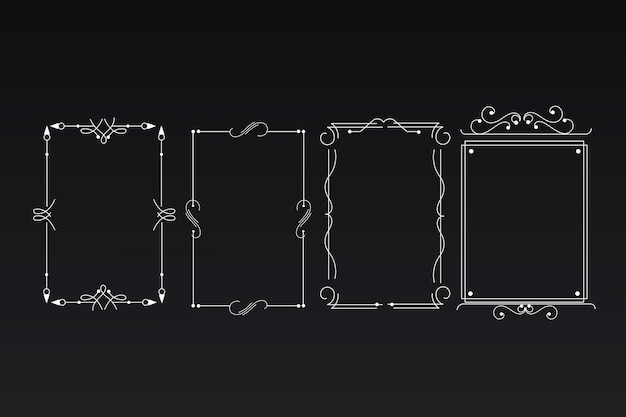The image features a completely black background with four elongated rectangular frames arranged side by side horizontally. Each frame is illustrated in detailed white ink, showcasing distinct and intricate patterns along their borders, but with no pictures or text inside. The frames are designed to inspire customization, perhaps for inserting personal photos or artwork, or even for use as an invitation template. The leftmost frame is bordered with pretzel-shaped patterns on the verticals and curvy shapes reminiscent of a uterus on the horizontals. The second rectangle features paper clip-like designs around all sides. The third frame incorporates a-heart shaped panel at the top, wing-like shapes on the sides, and two horizontal lines with an arched space in between. The rightmost frame combines wig-like patterns at the top and a shape resembling ovaries at the bottom, with the vertical edges defined by simple white lines. Despite their varying styles, the four frames share a uniform rectangular shape and a striking black-and-white color scheme, making each one unique yet cohesively part of the set.